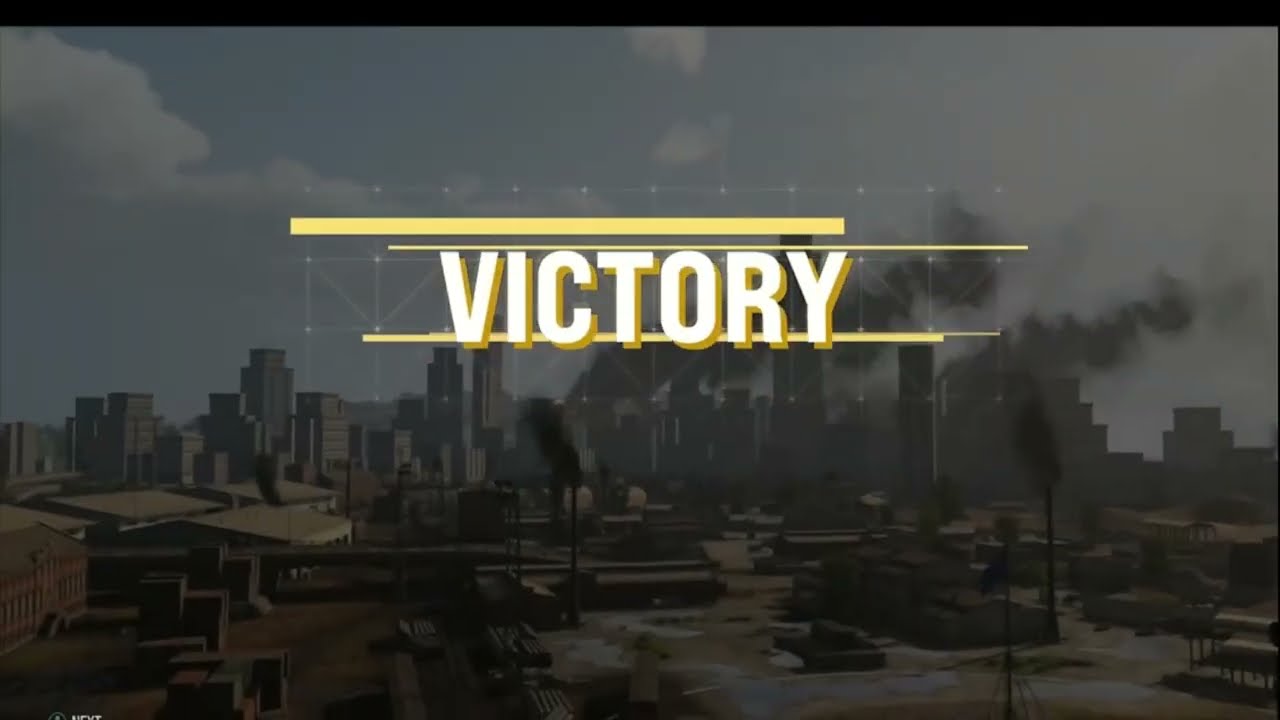This image appears to be a victory screen from a video game, vividly capturing the aftermath of a completed mission. Dominating the center of the image, the word "VICTORY" is prominently displayed in large white letters with a yellow border. Above and below the word are thick and thin tan stripes, adding to the celebratory design. The background reveals a cityscape under a grey, cloudy sky, with an ominous dark tint pervading the scene. Black smoke billows from smokestacks rising from several mid-sized buildings on the right-hand side, contrasting with the more orange and brown hues of the closer rooftops and smaller industrial structures. The city itself appears war-torn or heavily industrialized, with earth tones of black, brown, and tan giving the impression of a grim, rubble-strewn environment. Scattered trees and clouds complete the scene, evoking a sense of desolation despite the victorious message.